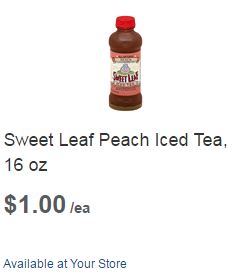The image features a product advertisement set against a completely white background, likely for an online store or flyer. Central to the image is a brownish plastic bottle labeled "Sweet Leaf Peach Iced Tea" with a distinctive red cap and a white and red front label. Below the product, the text details the offering: "Sweet Leaf Peach Iced Tea, 16 ounces." The price is prominently displayed in a larger, bold font as "$1.00," followed by "/EA" in a smaller font, indicating the price per unit. Further down, in a blue, different styled font, it states, "available at your store."